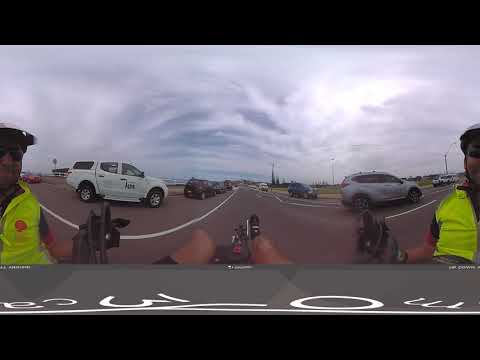The image captures a vertical, rectangular panoramic view featuring two individuals standing on opposite sides of a road, each wearing neon yellow or green vests with black helmets. The person on the left is partially visible, showing only their legs from the knees down, while the right side reveals more details, including a yellow vest with a red logo, a black helmet, and sunglasses. They appear to be facing opposite directions. The road itself is dark gray pavement marked with solid white lines and a horizontal white line extending towards a gray SUV positioned on the right, near the passenger side. Further vehicles include a white Suburban on the left and others scattered in the background, amidst patches of green grass and distant trees under a gray, cloudy sky. The image, possibly taken from a camera on a bicycle, has a black strip both at the top and bottom, and on the lower section, there are faintly visible alphanumeric characters, including an upside-down 'A,' a 'C,' '3,' '0,' or 'O,' and an 'M.' The overall scene suggests the photo has a filtered, slightly curved effect, emphasizing the staged or organized nature of the setting.